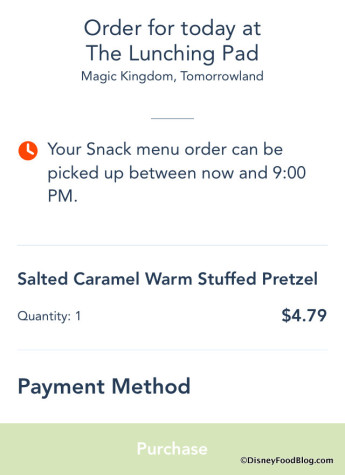Caption: 

The image features a mobile order confirmation screen from the Lunching Pad in Magic Kingdom's Tomorrowland. At the top of the screen, the text "Order for Today" is clearly displayed. Below this, there is a gap followed by a small red clock icon featuring two white hands on the left side, indicating the message: "Your snack menu order can be picked up between now and 9:00 PM."

A faint gray line separates sections of information. The text continues by listing the order details: "Salted Caramel Warm Stuffed Pretzel" with a quantity of one priced at $4.79. Another faint gray line follows, leading to the text "Payment Method" written in black on the left side of the screen.

The background of the lower part of the screen is light green. In white text on this light green section, the word "Purchase" appears, implying that the purchase can be confirmed by clicking on it, or it may indicate that the payment has already been made. In the bottom right corner of the light green area, a copyright symbol along with the text "DisneyFoodBlog.com" is written in a purplish color.